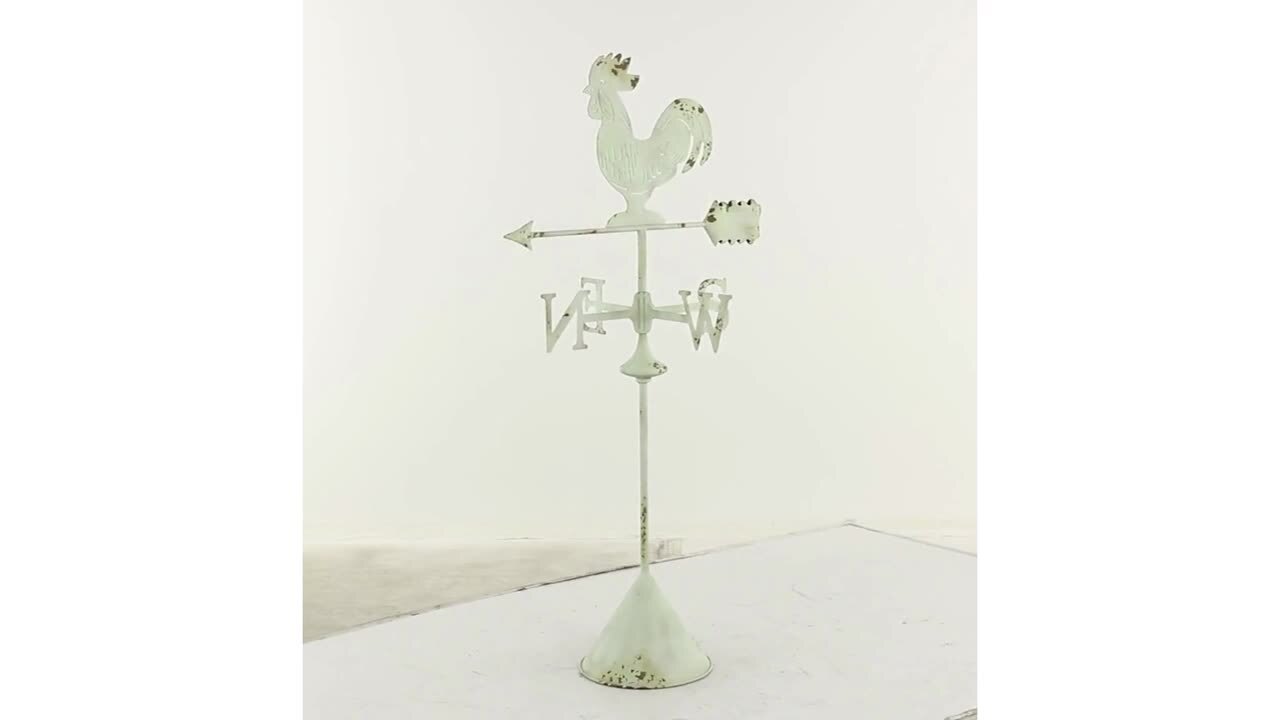This image captures a detailed side view of a weather vane, prominently centered in the photograph against a completely white, opaque background. The weather vane features a base shaped like an inverted cone, from which a rod extends upward. At the midpoint of the rod, directional indicators are visible, with 'N' for north pointing to the left and 'S' for south to the right. Perched on top of a horizontal arrow, which points left towards the north, is a rooster. The rooster, metallic and predominantly white with hints of black near its top, faces north with its tail towards the south. The entire structure, including the cone base and directional letters, appears metallic and exhibits signs of weathering, suggesting it has been well-used and exposed to the elements.